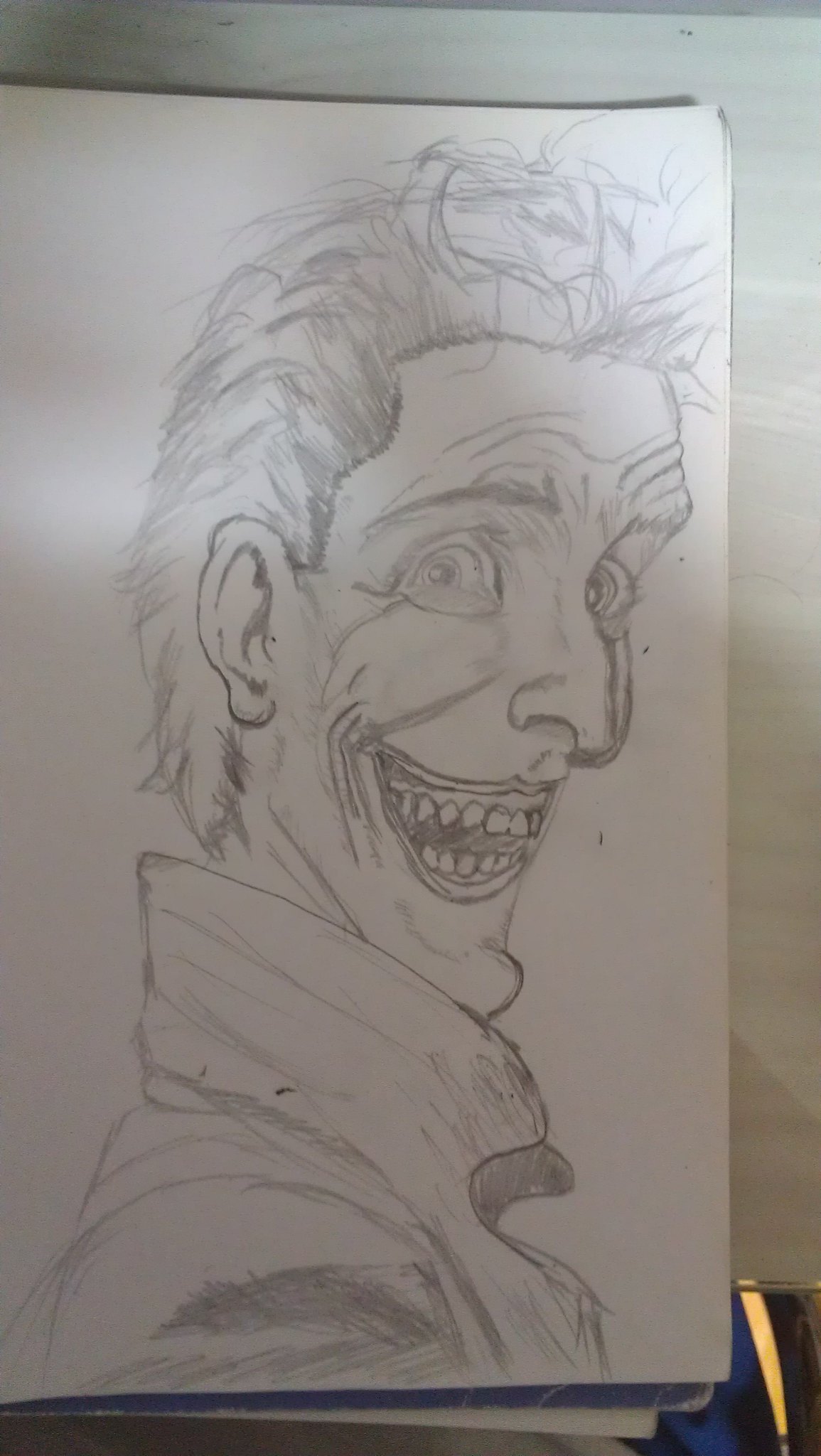This image showcases a detailed pencil sketch on a pristine white piece of paper, laid atop another sheet. In the lower right-hand corner, the top part of a sophisticated black and gold pen protrudes, hinting at the possibility that the artwork was created with this pen rather than pencil. The subject of the sketch is an intriguing blend of Ichabod Crane and the Joker from Batman. The figure is distinctly emaciated, embodying the eerie qualities of both characters. It features short, spiky hair on top, with spikes extending down the back, and an exaggerated, high-cut style around a prominent ear. The character’s sinister smile reveals crooked teeth, adding to its menacing aura. Completing the visage is a long, beak-like nose, enhancing the overall spooky and unsettling appearance.